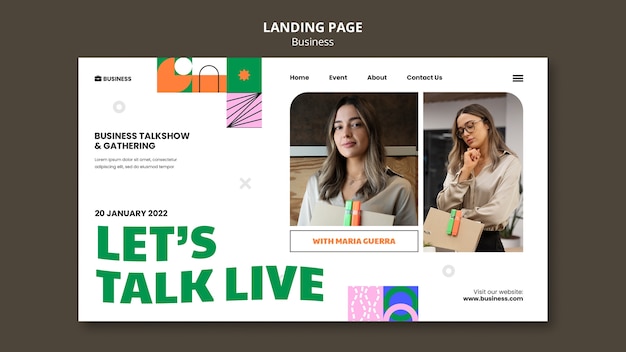A detailed caption for the given image description might read:

"This landscape-oriented screenshot captures a professional website template designed for building business or personal web pages. The outer edge is framed with a brown border containing white text that reads 'Landing Page Business'. Inside, against a white background resembling a typical landing page layout, the upper left corner features the word 'Business' followed by the subtitle 'Business Talk Show and Gathering.' The date '20 January 2022' is displayed beneath this in smaller text. Dominating the central area, large green curved letters proclaim 'Let's Talk Live'. 

On the right side of the image, two photographs of the same woman, likely Maria Guerra, are displayed. In the first image, she is shown with long brownish-blonde hair, wearing a beige button-up blouse, and holding a folder, possibly with highlighters attached. In the second image, she is wearing glasses and resting her head on her knuckles, looking downward. A text box beneath the images bears the caption 'With Maria Guerra'.

At the very bottom of her images, there appears a line of text, 'Visit our website www.business.com'. The top navigation bar of the page includes links labeled 'Home,' 'Event,' 'About,' and 'Contact Us,' alongside a hamburger menu icon in the upper right corner, suggesting additional options when clicked."